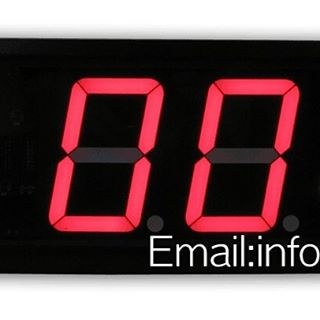This image features a close-up view of a digital display screen. Dominating the view is a single, illuminated square segment with a black background. The digital display itself shows the digits "00" in a soft, light red color. In the bottom right-hand corner of this segment, text appears in white font, reading: "email: info". There is no additional context or information provided, suggesting this could be a fragment of a larger digital interface. The lack of surrounding details leaves the purpose and broader context of the display ambiguous.